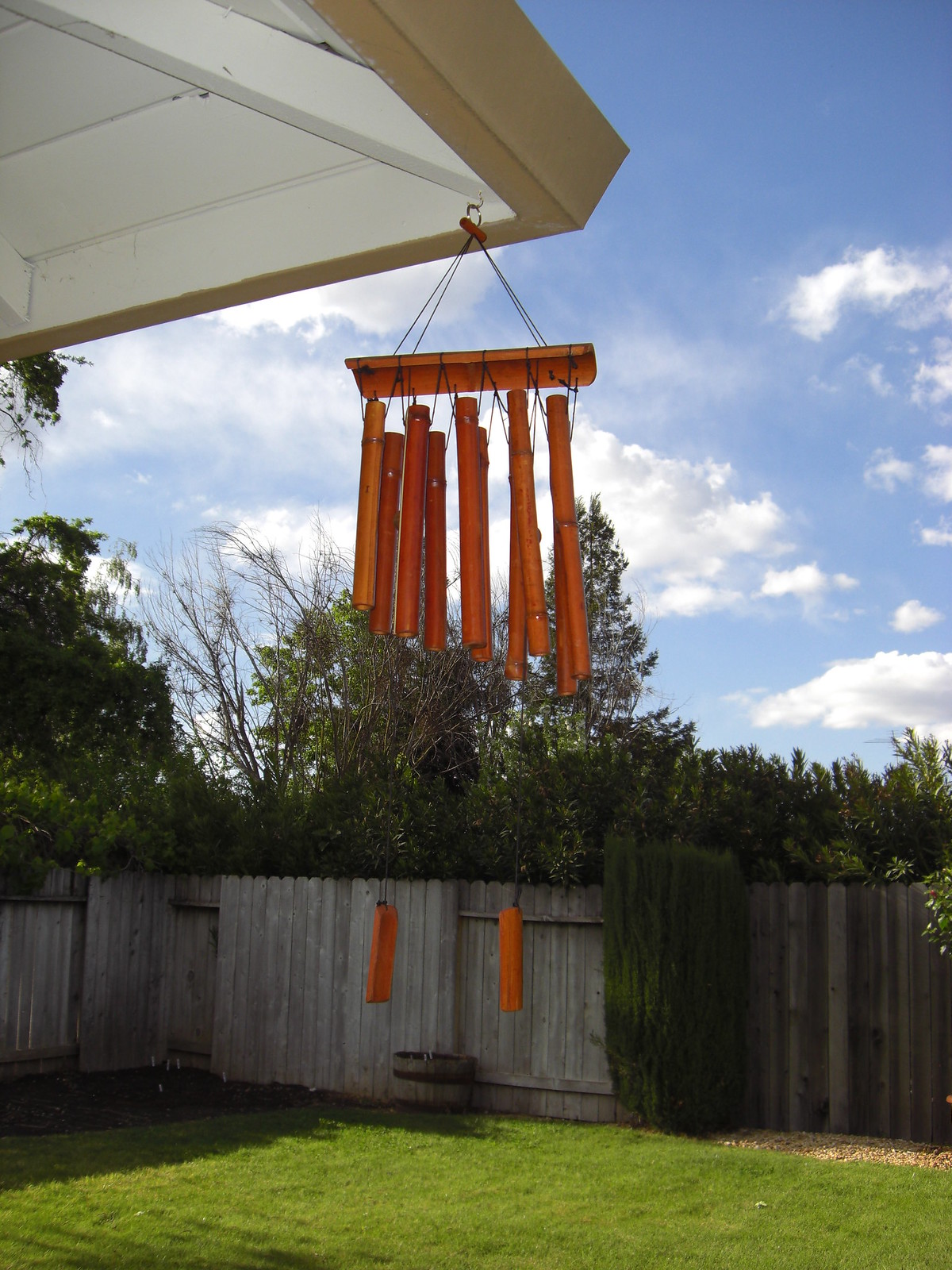This vibrant color photograph, taken in portrait orientation, captures a meticulously manicured backyard garden. The centerpiece of the image features a vivid orange wind chime with long tassels, hanging from a white plastic-paneled awning that extends horizontally to the left. The lush green lawn beneath is perfectly trimmed, indicating careful maintenance. 

In the bottom third of the image, along the edge of the lawn, a light tan brown wooden fence frames the scene, running across the back and at a 90-degree angle off the left-hand corner. In one corner of the lawn, there's a circular patch of brown mulch, potentially designated for planting. Some parts of the fence line are bordered with a line of decorative rocks, possibly marking the beginnings of a garden section with tall shrubbery.

Beyond the fence, a variety of trees and bushy shrubs, some adorned with dark green foliage and others bare, create a natural backdrop. In the distance, the blue sky is interspersed with fluffy wispy white clouds, suggesting a pleasant and sunny day. The description richly details both the focal wind chime and the serene garden setting, emphasizing the harmonious blend of natural and man-made elements.